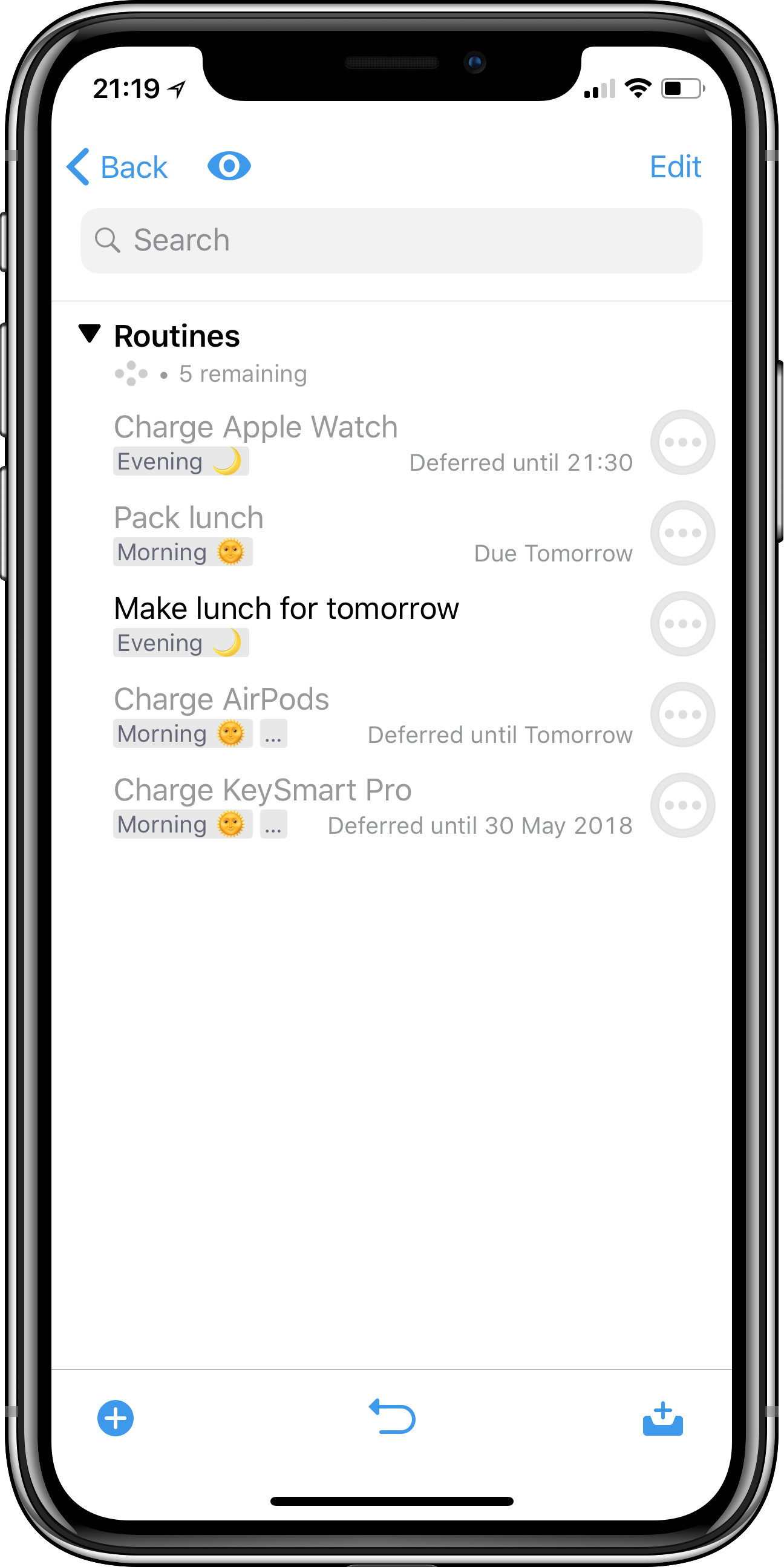This image displays an iPhone screen showcasing various scheduled tasks within a productivity app. At the top right corner, the indicators for network signal strength, Wi-Fi connectivity, and battery level are visible. The top left corner shows the current time. The interface lists several tasks and routines organized by specific times or events. Tasks include 'Charge Apple Watch' deferred until 21:30 in the evening, 'Pack Lunch' scheduled for the morning, 'Make Lunch for Tomorrow' due the next day, 'Charge AirPods' deferred until the following morning, and 'Charge KeySmart Pro' postponed until May 30, 2018. Each task is clearly labeled with its respective due time or status, helping to keep the user organized.